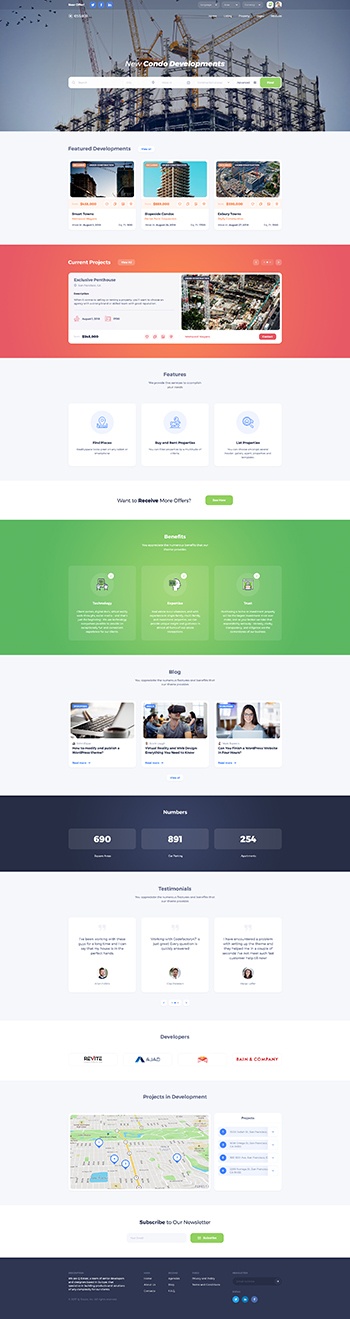The screenshot is viewed in portrait mode and appears slightly distorted. At the top, there's a title that reads "New Condo Developments" superimposed over a background photograph of ongoing construction. Below the title, a white search bar is prominently positioned.

Under the search bar, three rectangular images show buildings in different stages of construction, though they are slightly distorted. An orange rectangle follows, featuring another photograph of a construction site.

Beneath the orange rectangle, there is a section with white text and blue icons. This is followed by a green rectangle containing three boxes, each with icons and text.

Further down, three more photographs are displayed: one of a laptop, another of a person wearing virtual reality glasses, and the last of a woman using a laptop.

A navy blue rectangle containing text and numbers comes next in the layout. Below it are three white boxes featuring quotes and round avatar images.

Finally, at the very bottom of the screenshot, a map is displayed with four pins marking specific locations.